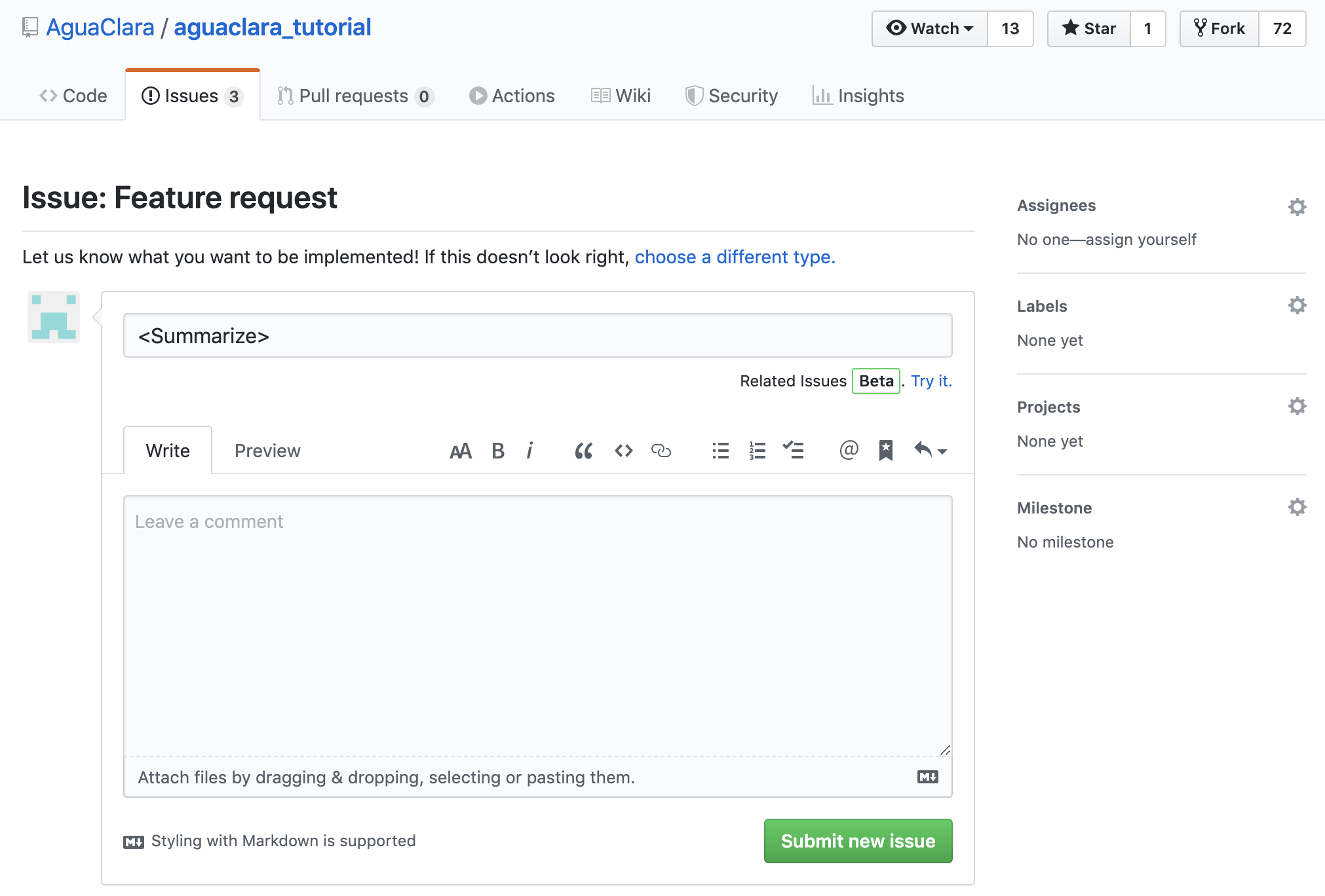**Caption:**

The screenshot showcases an application interface titled "Agua Clara / Agua Clara Tutorial," displayed on a computing device that could be a computer, tablet, or phone. In the top right corner, there are several icons and labels: a "watch" drop-down with an eye icon and the number 13, a "Star" label with an adjacent star icon and the number one, a "fork" icon with the label "Fork" and the number 72.

Below these, there is a row of tabs, which includes:
- **Code**
- **Issues** (with the number 3 and an exclamation point in a circle)
- **Pull Requests** (depicted with a pulley icon and a zero next to it)
- **Actions** (featuring a play button icon with a gray circle around it)
- **Wiki** (showcased with a book icon)
- **Security** (displaying a shield icon, half dark and half light)
- **Insights** (with a bar graph icon)

Under the "Issues" tab, there's an option to "open a feature request." The phrase "Let us know what you want to be implemented" encourages users to specify their requests. The clickable link "Choose a different type" is highlighted in blue, offering alternative options if the current type is unsuitable.

Below that, there's a suggestion to "Summarize in open and closed brackets" with a feature request space labeled "related issues" in beta, indicated by a green square and the clickable, blue-text "Try it."

Directly beneath is a text box for writing the request, flanked by two tabs: "Write" and "Preview," with the "Write" tab currently active. Additional instructions advise users to "leave a comment" and provide various methods to attach files.

The text editing tools include standard formatting icons: bold, italics, quotation marks, bullet points, and an "M" with a downward arrow which signifies that "Styling with Markdown is supported." At the bottom right, there's a green button with white text that reads "Submit new issue."